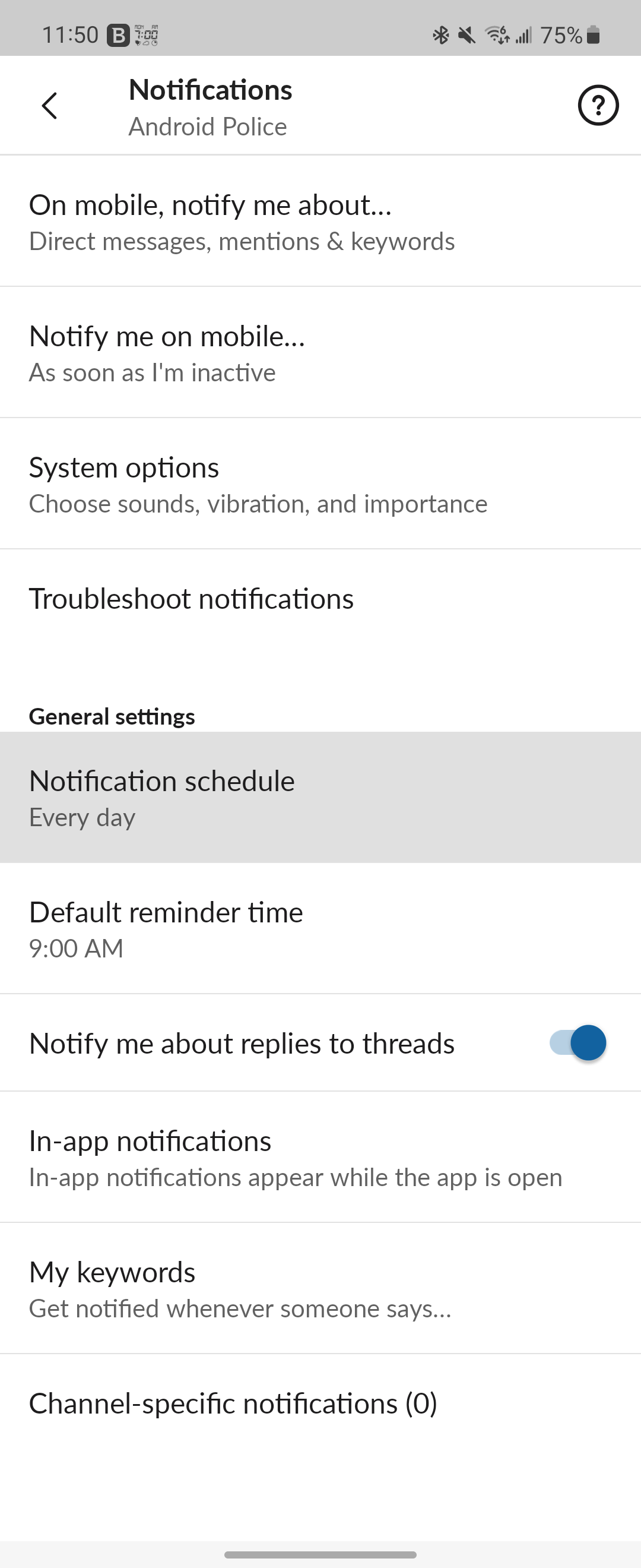In this image, we have a predominantly gray background at the top. On the left side, it reads "11:50" in gray text outlined in black. Adjacent to this are icons for Wi-Fi and a battery indicator showing 75% charge. To the left, there is a gray arrow pointing left and in black font, it reads "Notifications - Android Police." Next to this, there is a black circle with a black question mark inside.

The next section is titled "Notify me about." Under this heading, there are options for:
- Direct messages
- Mentions
- Keywords

Each option is separated by a gray line. Below, there's another line reading "Notify me on mobile..." followed by options for statuses such as:
- As soon as I am active
- I’m inactive

This is followed by another gray dividing line. The section "System options" includes the choices:
- Choose sounds
- Vibrations
- Importance

This is again divided by a gray line. Below that, a section titled "General settings" appears in smaller gray font.

In a gray box with a gray background and black font, it reads:
- "Notification schedule," set for "Every day"

This is followed by default reminder time info in a white background with black font:
- "Default reminder time: 9 a.m."

Following another gray line, there is text reading "Notify me about replies to threads" with a blue circle indicating this option is enabled to the right. Below this, another gray line leads to "In-app notifications." This states, "In-app notifications appear while the app is open."

The next section, divided by a gray line again, reads "My keywords." It explains, "Get notified whenever someone says..." and ends with an ellipsis.

Below, a final gray line appears, followed by the text "Channel specific notifications (0)" inside a gray box. The section concludes with a darker gray line through the middle.